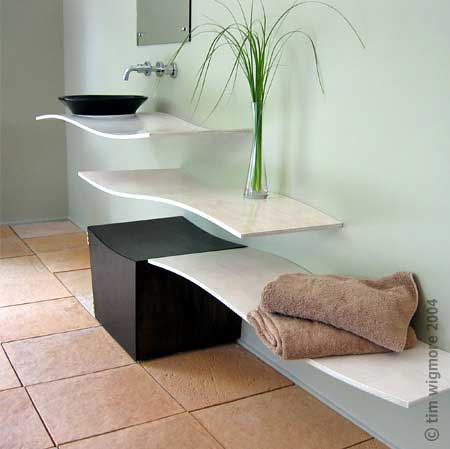The image showcases a thoughtfully designed bathroom with light seafoam green walls. Prominently featured is a minimalist setup devoid of traditional countertops. On the right side, a mirror partially reveals the wall and the unique faucet design. The faucets, embedded directly into the wall, hover above a sleek, large, black round sink basin. The basin is seamlessly integrated into a wavy, white countertop that securely holds it in place.

Descending from the sink area, there's a clever use of space: a secondary wave-like countertop supports a large glass vase. The vase, thick at its base and tapering gracefully towards the top, is filled with long, green stems resembling blades of grass.

Below this, a tall black stool aligns perfectly under the sink area, nestling into the diagonal arrangement of the wave-like shelves. On the third shelf, two light brown towels are neatly folded, adding a touch of warmth and texture to the cool green and monochrome palette. The bathroom floor is laid with medium light brown tiles, grounding the room with a natural, earthy tone.